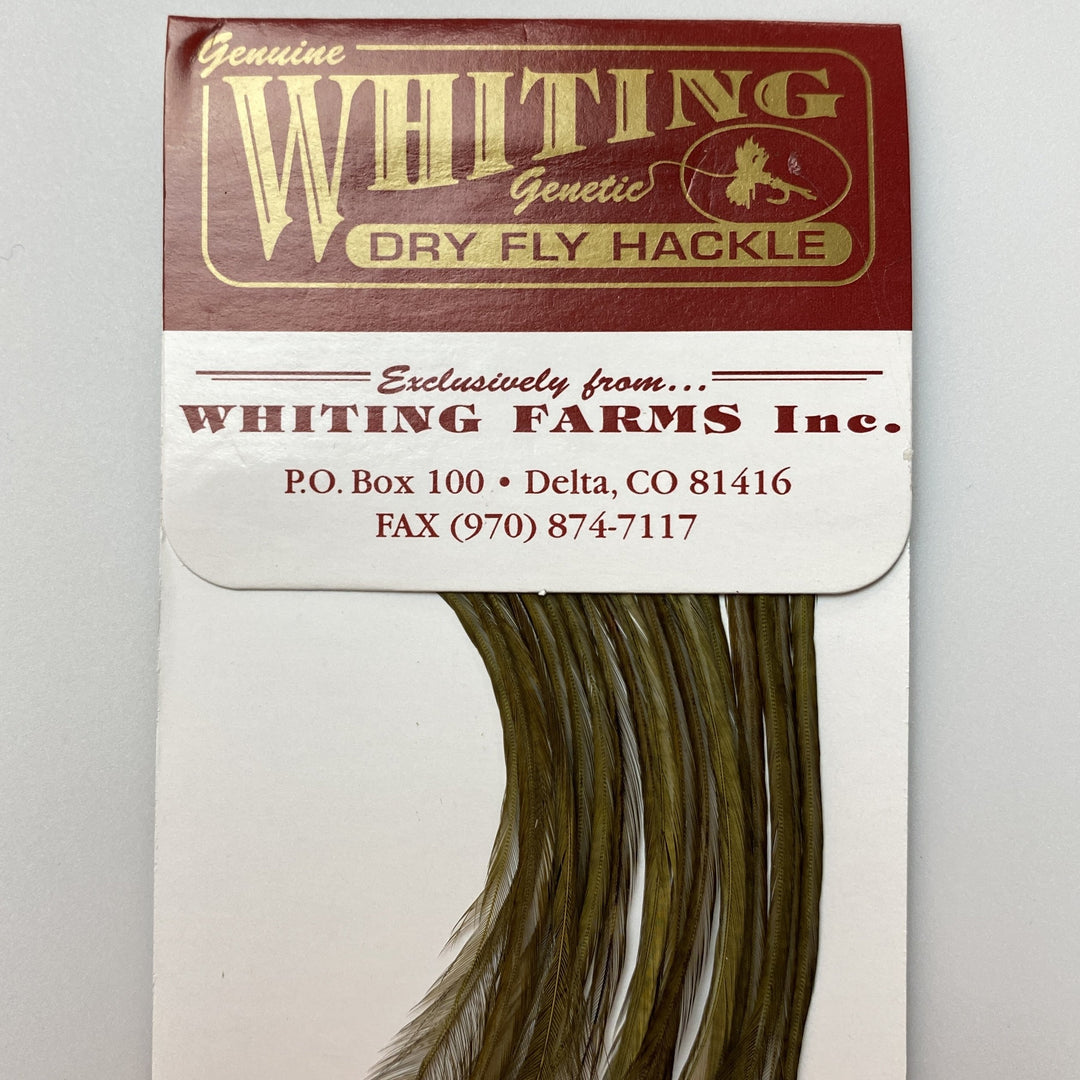The image features a product photo of Whiting Farms' dry fly hackle feathers, specifically designed for fly fishing. The feathers, around 15 in total, are meticulously rolled and enclosed in a distinctive package. The packaging consists of a white envelope with a striking red top section. In the red portion, there is elegant gold text stating "Genuine Whiting Genetic Dry Fly Hackle," accompanied by an illustration of a fly fishing lure connected to a fishing rod string. Below this red and gold section, the lower white portion bears a centered red text that reads "Exclusively from Whiting Farms Incorporated, P.O. Box 100 Delta, Colorado 81416" along with their fax number. The feathers inside are a key component for creating a snapping sound at the end of a whip, emphasized by their precise arrangement.